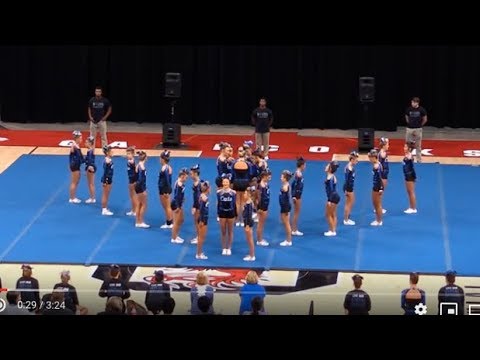This image captures a team of cheerleaders in a vibrant, dynamic scene as they prepare to begin their performance at a competition held in a stadium. The cheerleaders, donned in blue uniforms with white sneakers and white bows in their hair, stand poised on a large, blue rectangular mat. Their formation is primarily a triangular or V-shape, with some members in a circular group in the center, seemingly ready to execute a lift. Surrounding the stage, a black curtain hangs to the top of the image, while a vivid red border adds a splash of contrast. The presence of judges seated toward the bottom of the image, coupled with individuals in black shirts and tan pants standing behind the team, suggests the organizational structure and official nature of the event. Further in the background, other cheerleaders, coaches, and spectators are visible, highlighting the competitive and supportive atmosphere. The venue itself hints at a sports auditorium, possibly a school, with features like a light brown wooden basketball court beneath the mat and red accents with white lettering, affirming the energetic ambiance of the scene.